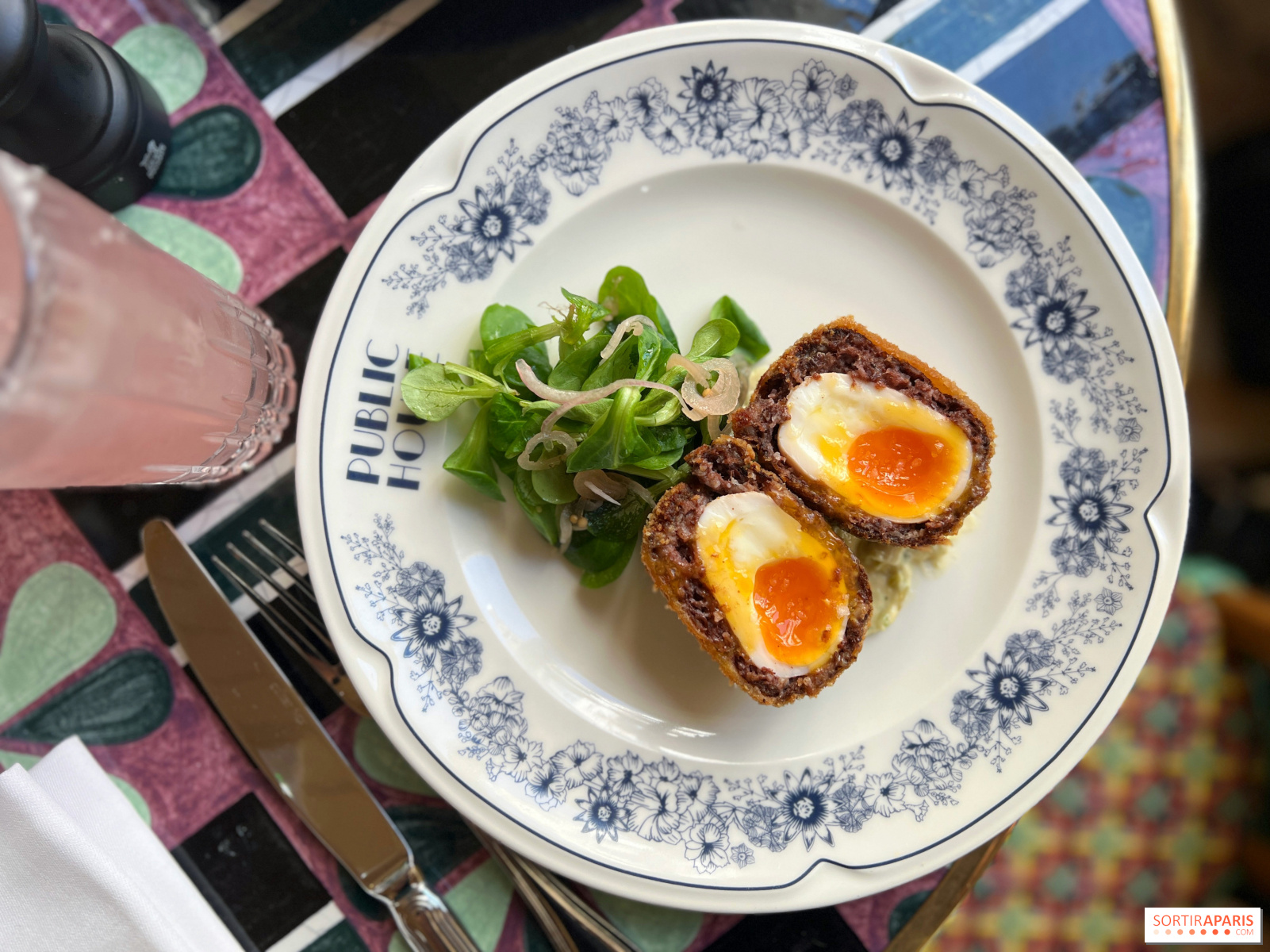A top-down view reveals a white plate adorned with a blue floral design along its border and the words "Public House" partly visible through a small green leafy salad near the top. The plate features two jammy, bright orange-centered fermented century eggs, each encased in a brown fermented layer. The eggs are garnished with green leaves and a bit of onion. Accompanying the dish, a glass of pink lemonade stands to the far left, while a metal knife and fork rest nearby on placemats.